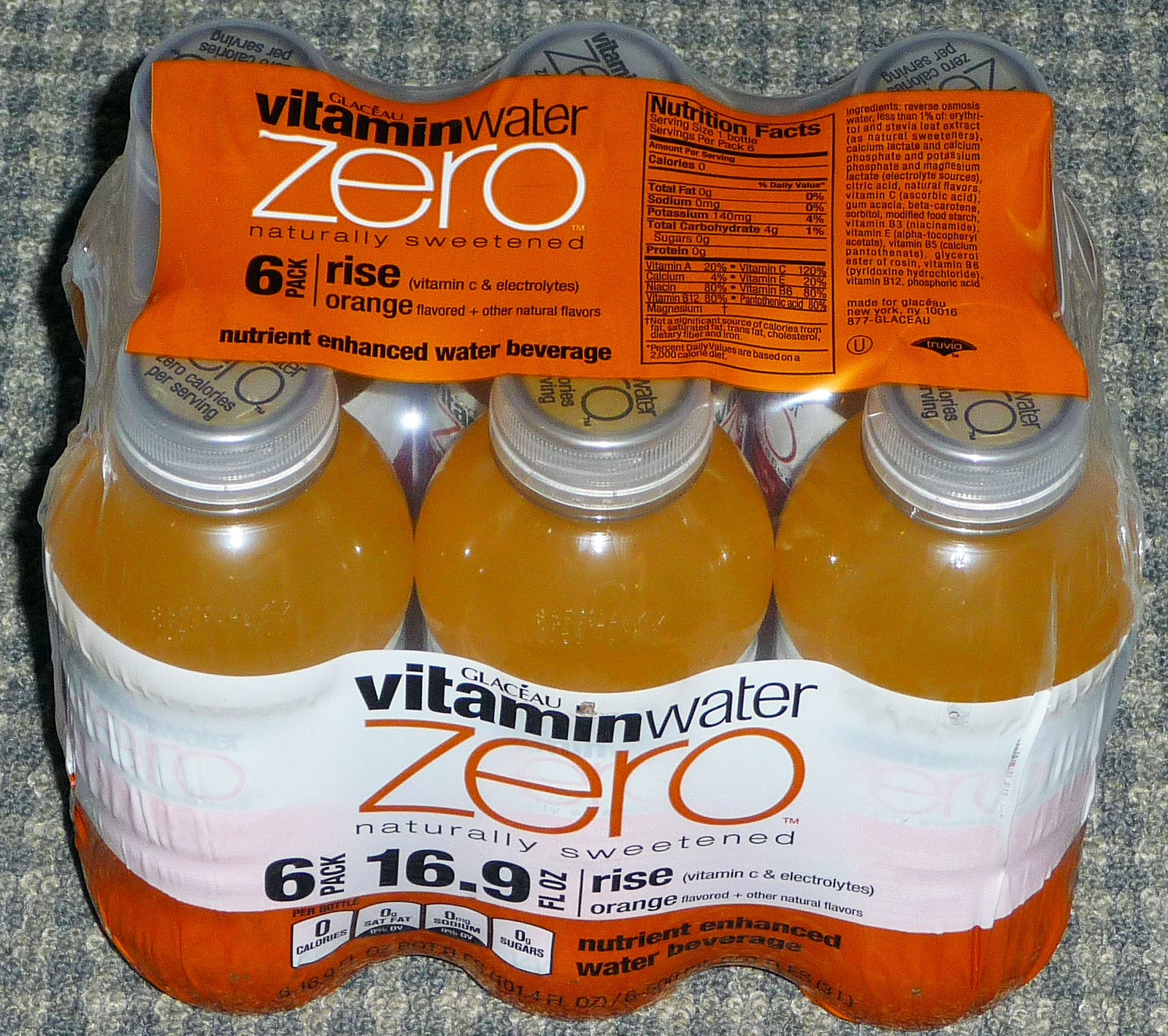This photograph presents an overhead view of a six-pack of Glacéau Vitamin Water Zero, specifically the "Rise Orange" flavor. The drinks are wrapped in transparent plastic packaging, allowing a clear view of the top and front sides of the pack. Prominently displayed on the top of the packaging is the brand name "Glacéau vitaminwater zero," with "vitamin" in bold black text and "zero" in smaller white text. Beneath this, the label reads "naturally sweetened six-pack." 

The packaging also indicates that this is a "nutrient enhanced water beverage." Adjacent to the central label, the nutritional facts are visible, detailing the calorie content along with the amounts of fat, sodium, potassium, carbohydrates, and sugars contained in the drink. Three of the bottles are prominently visible within the packaging, showcasing their distinct orangish-yellow color, while the remaining three are partially obscured. 

On the front of the pack, the label reiterates "vitaminwater zero" with "six-pack" clearly displayed. This front label stands out on a white background, with the word "zero" highlighted in orange text, aligning with the flavor's color scheme.